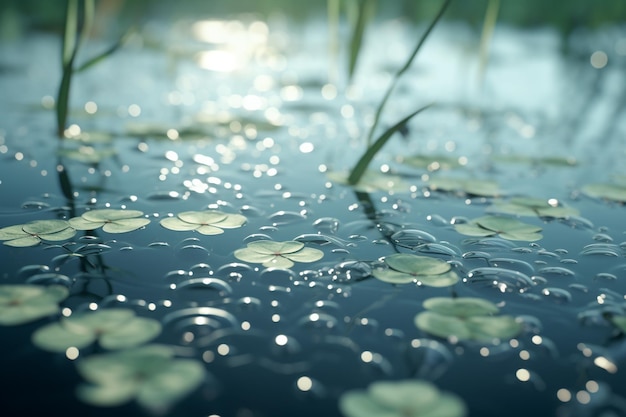This detailed close-up image captures the serene surface of a pond, characterized by a dark, deep blue hue. Prominently featured are a cluster of floating plants resembling clover, each with four or five overlapping leaves. Approximately 10 to 15 of these green clover-like plants are interspersed across the pond’s surface. Several blades of grass also pierce through the water, accentuating the natural green elements against the dark background. The surface is dotted with numerous light-reflecting bubbles, adding a sparkling effect to the scene. At the top right corner, a single white dot stands out, while a dozen more white dots line the lower edge in the foreground. The background of the image is blurred, contributing to a limited depth of field, with a subtle white patch suggesting an out-of-focus light source. The composition highlights the intricate beauty of the pond, focusing on the interplay of plant life and light reflections.